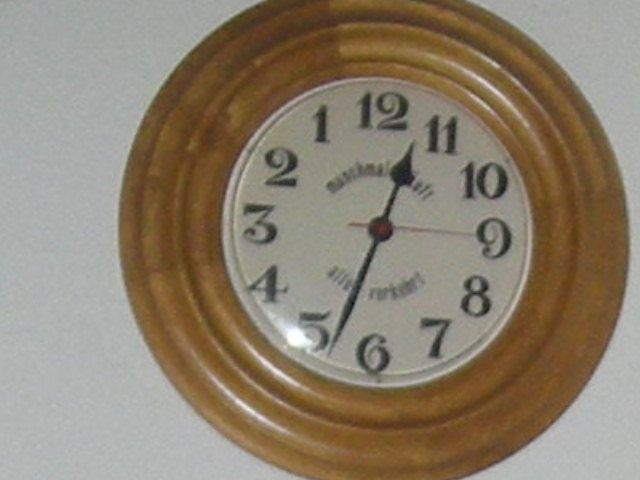This photo features a wall clock mounted on a white drywall surface. The clock has an oak-colored wooden frame, giving it a traditional, rustic appearance. Its white clock face is adorned with numerals in a curly, decorative font, beginning with '12' at the top. The time-telling hands consist of black hour and minute hands, contrasted by a red second hand. Despite the image being slightly out of focus, two sections of text are visible on the clock face — one located below the '12' and another above the '6', both in cursive script, likely indicating the brand name.